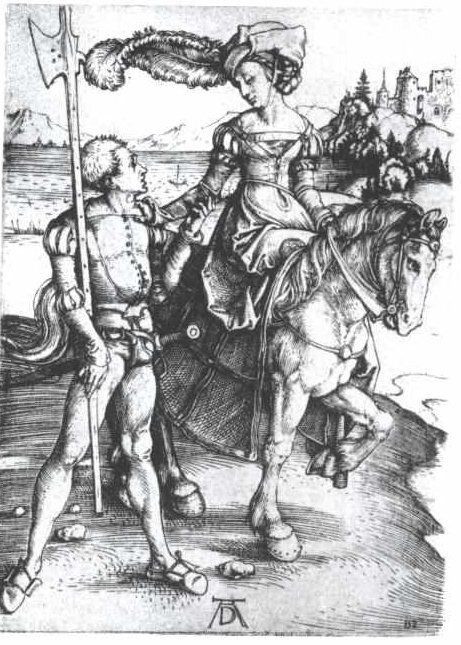In this captivating black-and-white illustration, a woman sits side-saddle on a muscular horse, which has its left front leg raised and head arched. She dons an ornate dress with billowing sleeves and a large, feathered hat that whispers in the wind. The woman adoringly looks down at a knight standing beside her, who, in turn, gazes up with affection. She reaches down with her right hand to touch his shoulder, while he gently grasps her elbow with his left hand. The knight is dressed in a suit of armor but with no helmet, and holds a large spear-like weapon in his right hand. Behind this romantic duo, a serene lake with a small boat stretches out, and beyond the lake, distant mountains rise majestically. In the upper right corner, a road leads to a medieval village, featuring a castle wall and a church, adding to the timeless charm of the scene.